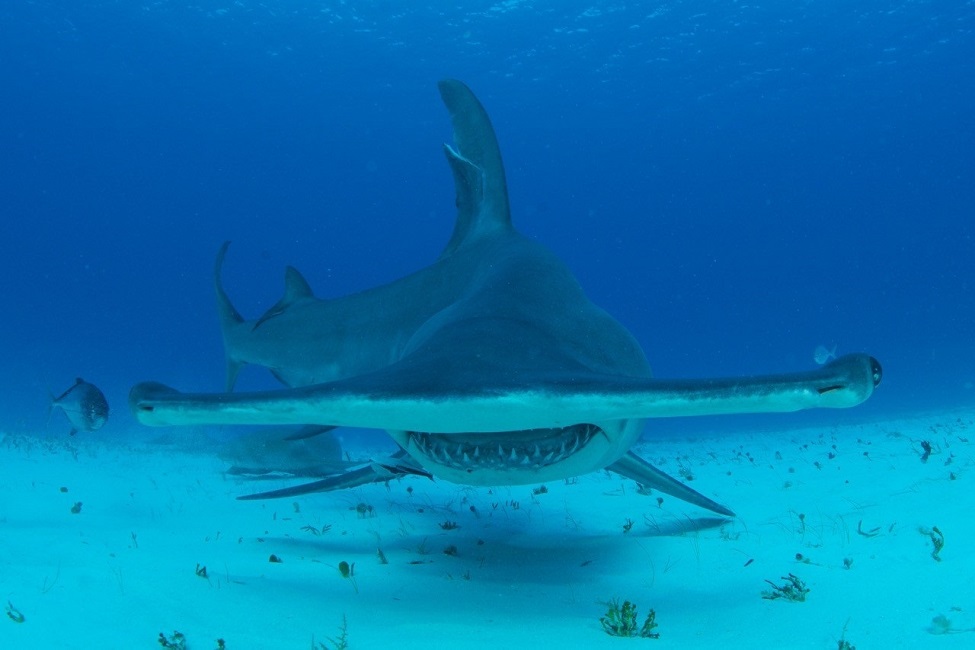This underwater photograph showcases a hammerhead shark swimming close to the ocean floor, amidst a backdrop of the blue water that transitions from darker hues above to lighter, almost greenish tones near the sandy bottom. Dominating the scene, the shark's distinctive, broad hammer-shaped head is seen head-on, with its black eyes positioned on either end of the hammer. Its mouth is open, revealing rows of sharp, pointy white teeth. Along with its formidable head, the shark’s body features a combination of white and gray coloring, with pronounced fins including a tall dorsal fin and a large tail fin. The ocean floor below is dotted with small green plants and a visible metal pole lying on the sand, seemingly about to be investigated by the shark. To the left of the shark's head, a smaller fish swims near its eye, adding to the vibrant underwater tapestry.